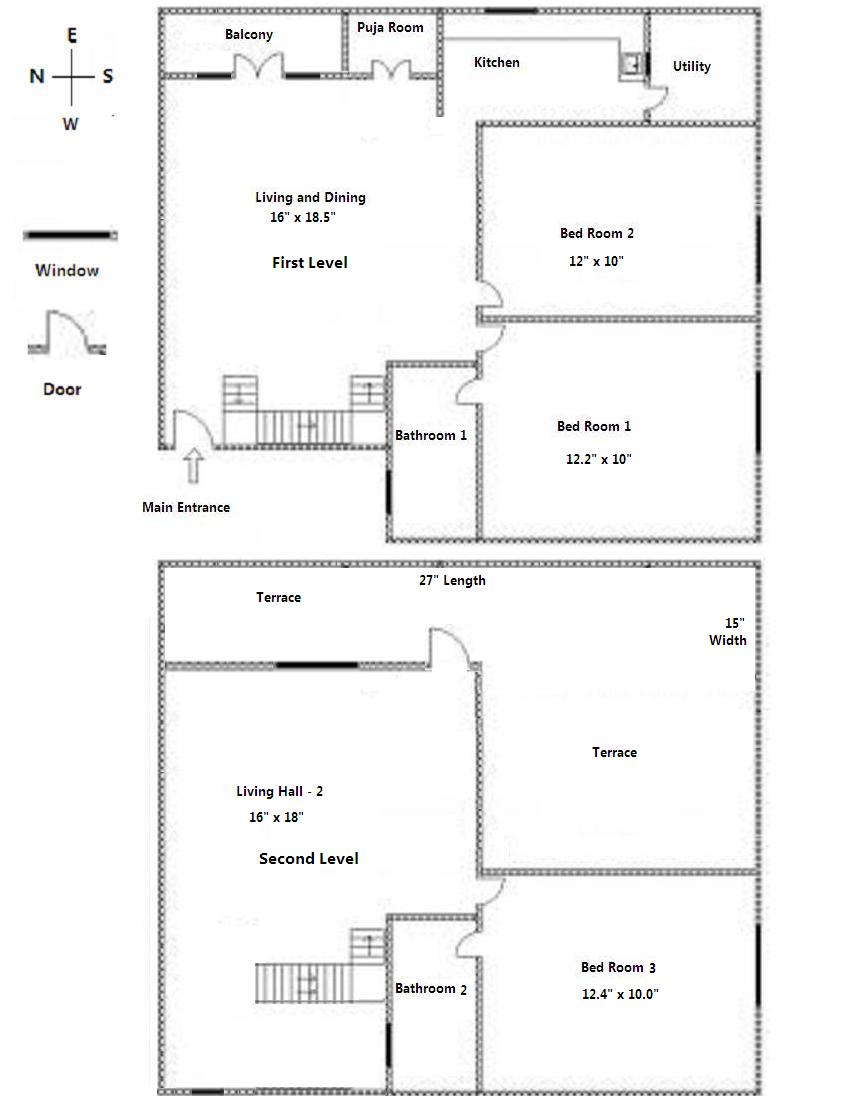The provided image is a black and white floor layout of a two-story house, detailing the arrangement and specifications of different rooms and features.

**First Level:**
- **Main Entrance:** Indicated by an arrow pointing towards a circular line located at the bottom left corner.
- **Open Space:** Right past the entrance, there's a large open area labeled "Living and Dining," measuring 16 feet by 18.5 feet.
- **Rooms and Areas:**
  - **Balcony:** Accessible space labeled as such.
  - **Pooja Room:** Situated adjacent to the balcony.
  - **Kitchen:** Positioned next to the Pooja room.
  - **Utility Area:** Located just below the kitchen.
  - **Bedroom 1:** One of the two bedrooms on this level.
  - **Bedroom 2:** The second bedroom on this level.

**Second Level:**
- **Terrace:** Main feature of the second floor, labeled twice, with dimensions of 27-inch length (possibly an error, likely feet), 24 feet in length, and 15 feet in width.
- **Bedroom 3:** A room with dimensions of 12.4 feet by 10.0 feet.
- **Living Room-2:** Another open living area on this level, measuring 16 feet by 18 feet.
- **Stairs:** Indicated by lines with two arrows pointing upward and another arrow pointing to the other side.

**Additional Features:**
- **Directional Compass:** On the left side of both floor plans, there's a cross with "E" at the top, "W" at the bottom, "N" on the left, and "S" on the right.
- **Windows:** Represented as a black bar.
- **Doors:** Illustrated as a bar with a break in the middle and a rounded section.

All details are illustrated in a monochromatic scheme, providing clarity on the spatial arrangement and measurements of the house's features.